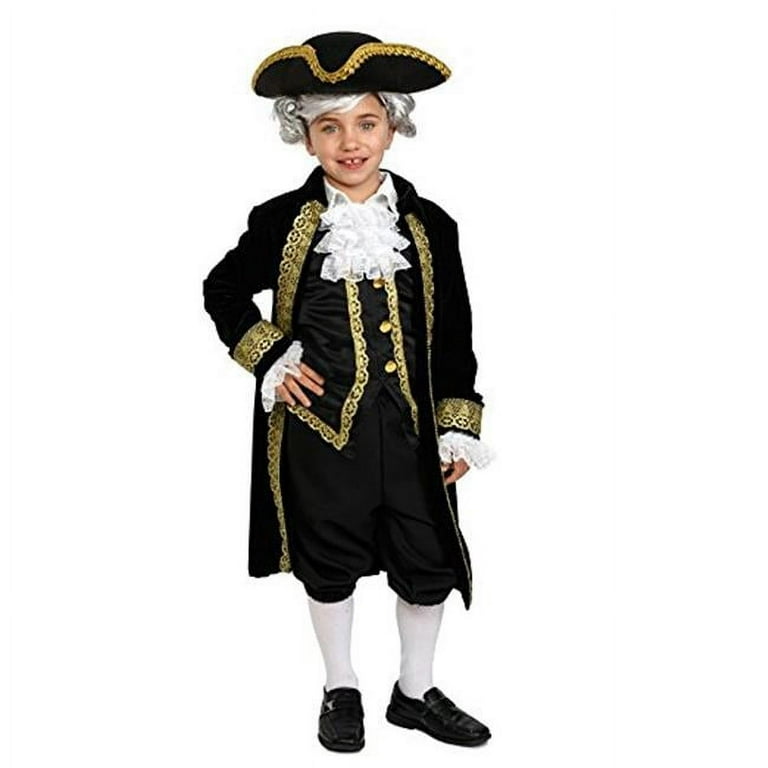In this indoor color photograph, a young boy, approximately six or seven years old, is captured in a close-up shot against a clean white background. The scene highlights his elaborate colonial-era costume, reminiscent of a Founding Father. The boy sports a silvery gray wig topped with a black tricorn hat adorned with gold trim, which matches the detailed gold banding on his dark overcoat. The overcoat features white ruffles at the sleeves, complementing his black pantaloons and white tights. His dark shoes complete the ensemble. The boy's right hand rests confidently on his hip as his left arm hangs by his side. He beams a toothy, gap-toothed smile directly at the camera, exuding happiness. The image likely serves to showcase or advertise the intricately designed costume.